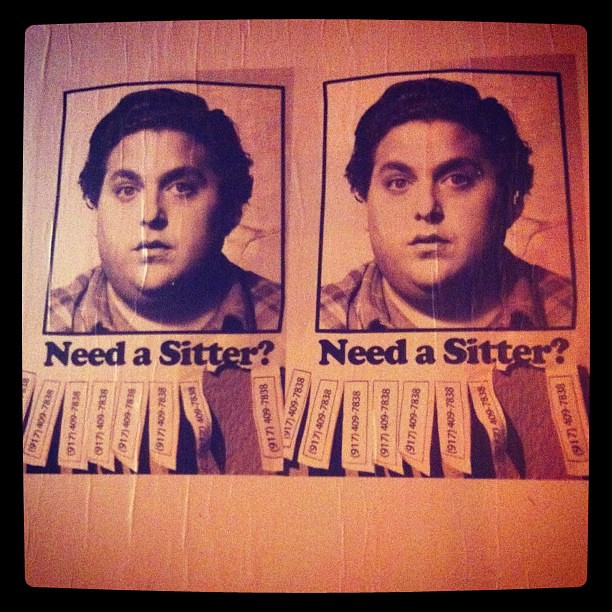The square photograph depicts a vintage-style advertisement, seemingly printed at home, featuring a twice-repeated image. The advertisement showcases a young man with dark wavy hair and a round face, resembling Jonah Hill, wearing a plaid collared shirt. Each image is encased in a black border, beneath which appears the bold text "Need a Sitter?". Multiple tear-off tabs with phone numbers are attached below the text, though some tabs have been removed. The dual images are arranged side-by-side, giving the impression of a bulletin board flyer. White lines run through the entire photograph, suggesting it has been pasted onto a textured surface, like a wall. The area below the pull-tabs remains white, reinforcing the homemade and aged appearance of the advertisement.